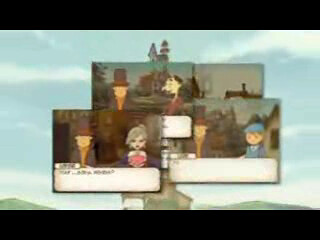The image appears to be a screenshot or photograph taken from a video game or piece of digital art. It features a scene framed by a thick black border at both the top and bottom. The background consists of a bright blue sky punctuated by small, white clouds, and there's a suggestion of mountains toward the bottom. Central to the image is a brown wooden house or castle with a large white door. 

Overlaying this scenic backdrop are four smaller squares, laid out in a collage-like fashion. These squares depict individuals in various settings:

1. The first square shows a man wearing a tall dark top hat, a brown turtleneck, and a brown jacket. He is sitting at a white table beside a woman dressed in pink, with her hair styled in a top knot bun.
2. The second square also features the same man in the tall dark hat, but this time he is accompanied by another individual, a man with thin brown hair and a notably long nose. 
3. In the third square, the man in the tall dark hat is seen again, this time with a boy dressed in blue, complete with a blue newsboy cap.
4. The fourth square is less distinct, showing primarily the blue sky without any discernible figures.

The overall effect is a somewhat blurry collage, combining individual portraits against a backdrop of nature, combining elements from video game imagery and traditional art styles.